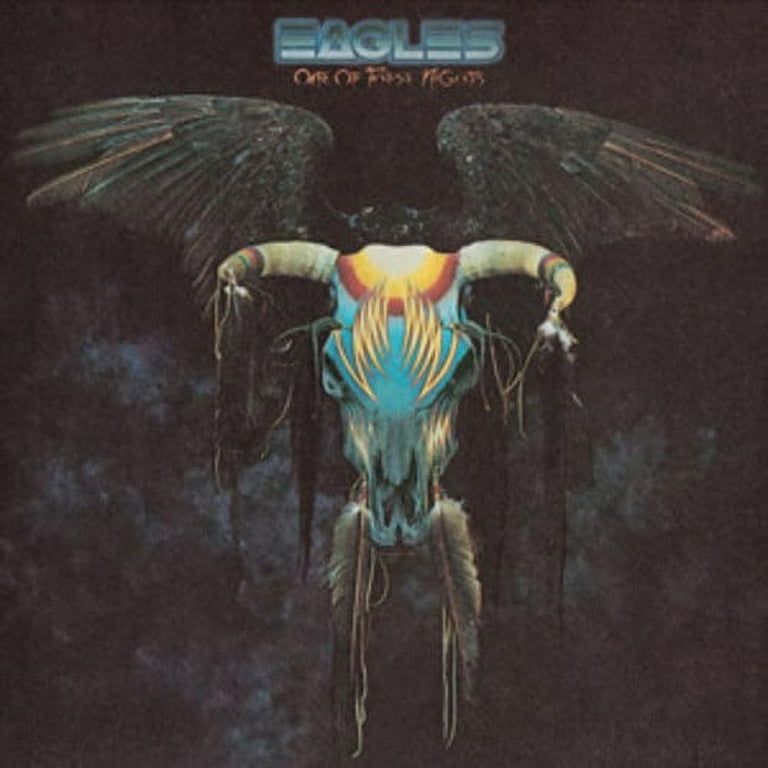This image is an album cover characterized by its pixelated and grainy appearance. At the top, in futuristic gradient text transitioning from dark to almost white, the cover prominently displays the name "Eagles." Below it, in smaller, slightly blurry orangish-red text, is the album title, difficult to decipher but possibly reading "Omen of First Nights."

The background is primarily black, fading into a silvery blue, smoky pattern towards the bottom, giving the image an aged and mystic feel. The central figure is a surreal, humanoid form, merging elements of an ox’s skull and angelic features. The skull is painted blue with a distinct design on its forehead comprised of concentric circles - a white center, encircled by yellow, and then a red border, resembling a yarmulke. Lightning-like patterns accentuate the skull’s features by the eyes and cheekbones.

The horns, facing forward, are adorned with rings of red, yellow, and green near their tips, and from them dangle strings and feathers, contributing to a Native American aesthetic. The figure’s large, black, and gray wings with light brown accents stretch out dramatically, enhancing its ethereal, otherworldly appearance. The body transitions into feather-like legs, and occupying the torso area is a devilish face with animalistic eyes and a butterfly-shaped mouth. The overall composition evokes a mix of mythological and futuristic elements, creating a hauntingly unique and detailed visual.